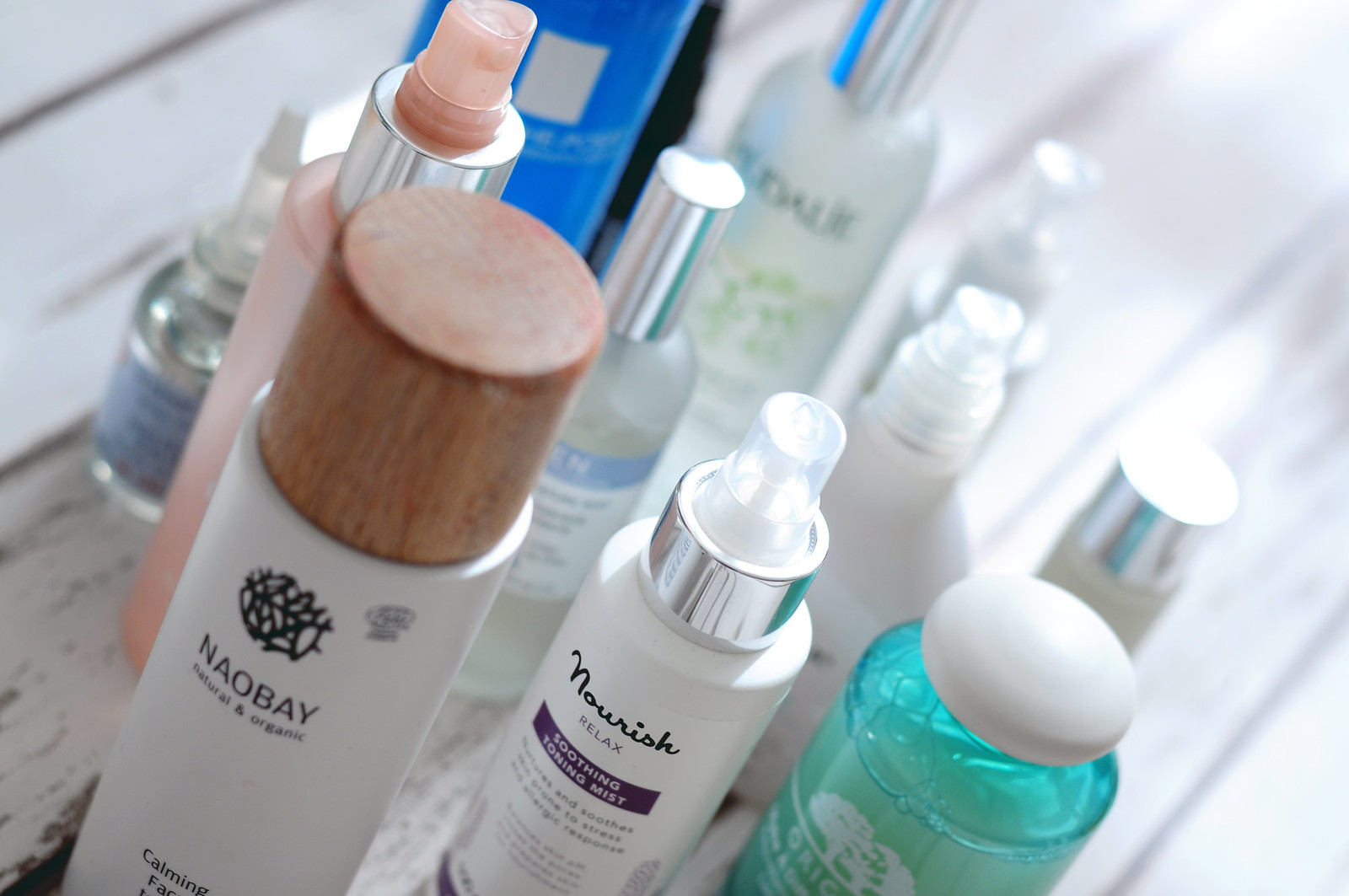This image showcases an assortment of skincare and personal health products, primarily focused on facial care. The items are neatly arranged on a surface that appears to be whitewashed wooden planks, contributing to a rustic and serene aesthetic. Central to the image is a green Origins bottle with a white cap, partially filled with a liquid that has a bubbly appearance at the top, giving the impression of a refreshing toner or serum.

Next to it stands a sleek white bottle with a silver rim and a small plastic cap, labeled "Nourish Relax Soothing Toning Mist." The bottle features the brand name "Nourish" in black, while "Relax" is highlighted in purple, accompanied by a delicate purple emblem, suggesting a calming and soothing product.

Adjacent to the Nourish spray is a white bottle with a wooden top, branded "Nail Bay." The visible text reads "Calming Face," indicating a product designed to soothe and pamper the skin. Additionally, the background holds several clear bottles crowned with silver tops, hinting at an array of serums or toners. There is also a partial view of a blue bottle, adding a pop of color to the arrangement.

The collection includes various pump and spray bottles, indicating a range of application methods tailored to different skincare routines and preferences.